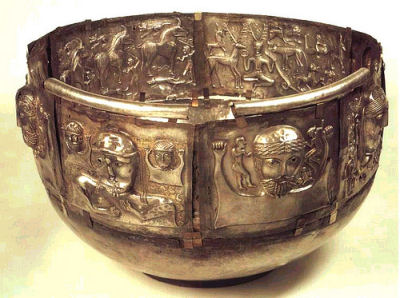This image depicts an ornate metallic bowl, likely brass or bronze, resting on a beige surface. The bowl’s exterior features an array of intricate engravings, illuminated by an overhead light that accentuates its golden hues, darker at the bottom and lighter towards the top. Prominent on the bowl’s exterior are several detailed faces characterized by curly hair, beards, and helmets, reminiscent of ancient Greek or Roman artistry. These faces appear in different sections around the bowl, interspersed with various other figures and motifs, including a man with his arms raised, a meditating individual, a dog, a deer, and three horses. The background of the image reveals a plain white wall, situating the scene indoors.